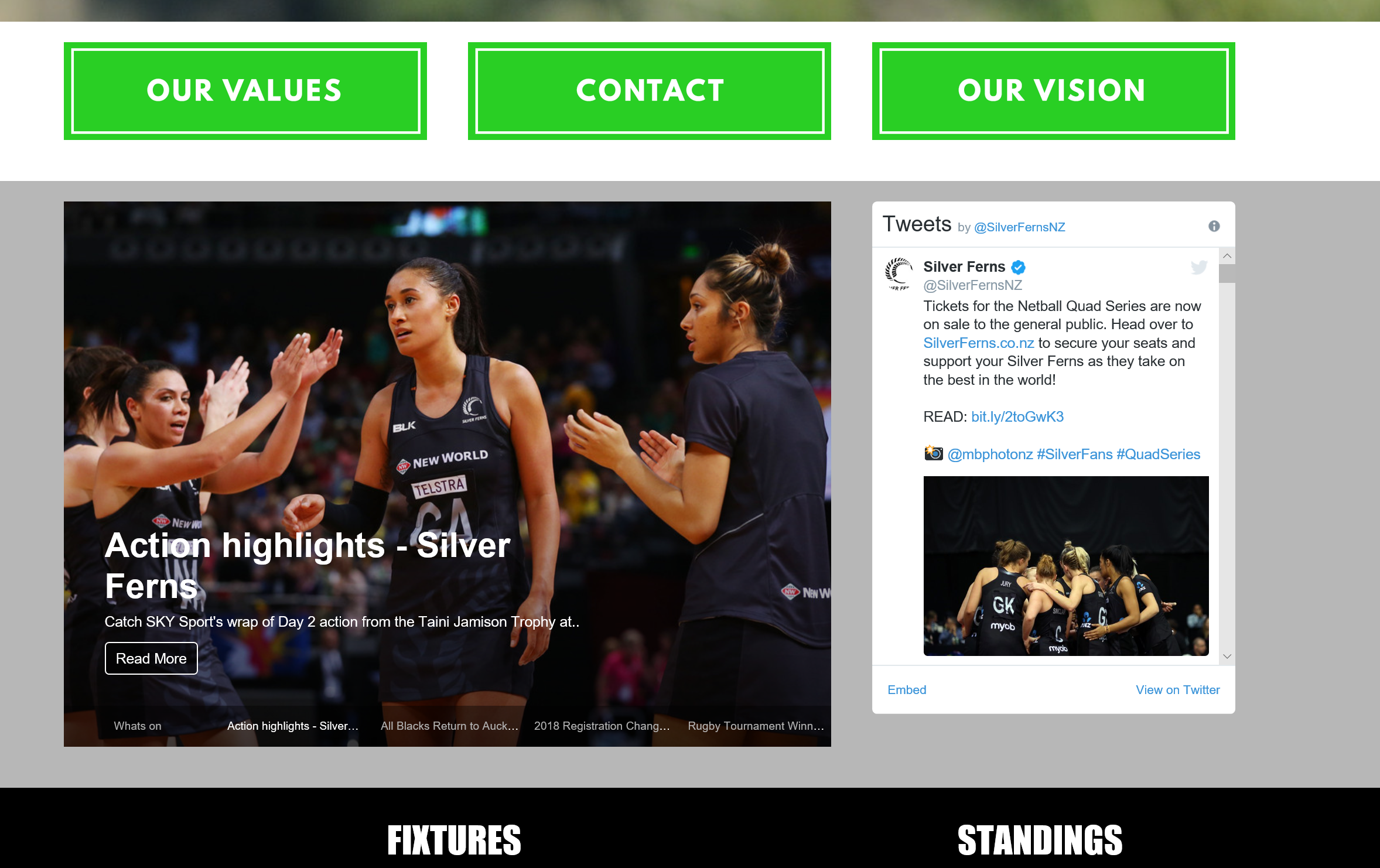The image description is as follows:

At the top of the image, there is a horizontally-oriented rectangle transitioning in color from gray to dark green, then to lighter green, light gray, back to green, gray, and green multiple times. Within this complex color pattern, there are three green rectangles, each with a white-outlined inner rectangle containing the following texts respectively: "Our Values," "Contact," and "Our Vision."

Below this section, there is a large gray rectangle occupying the central portion of the image. On the right-hand side of this gray section, there is a photograph depicting several women clapping, who appear to be wearing team uniforms. The text "Action Highlights - Silver Ferns" is displayed next to the image, with some small, unreadable white text beneath it. A button, which is either blue or black in color and outlined in white, labeled "Read More" is also present.

On the right-hand side of the gray rectangle, there is a white rectangle with the heading "Tweets" at the top. The text "By" is followed by a blue handle that is not clearly readable. Below this handle, there is a symbol resembling a feather, a check-marked blue circle, and the title "Silver Ferns." Further below, there is black and blue colored text with the word "Read" in black followed by unreadable blue text. This section also contains a small, indistinguishable picture with accompanying blue text, an additional image of the team, and two blue words positioned at the bottom left and right corners of the white rectangle.

At the bottom of the image, there is a black rectangle labeled "Fixtures and Standings."